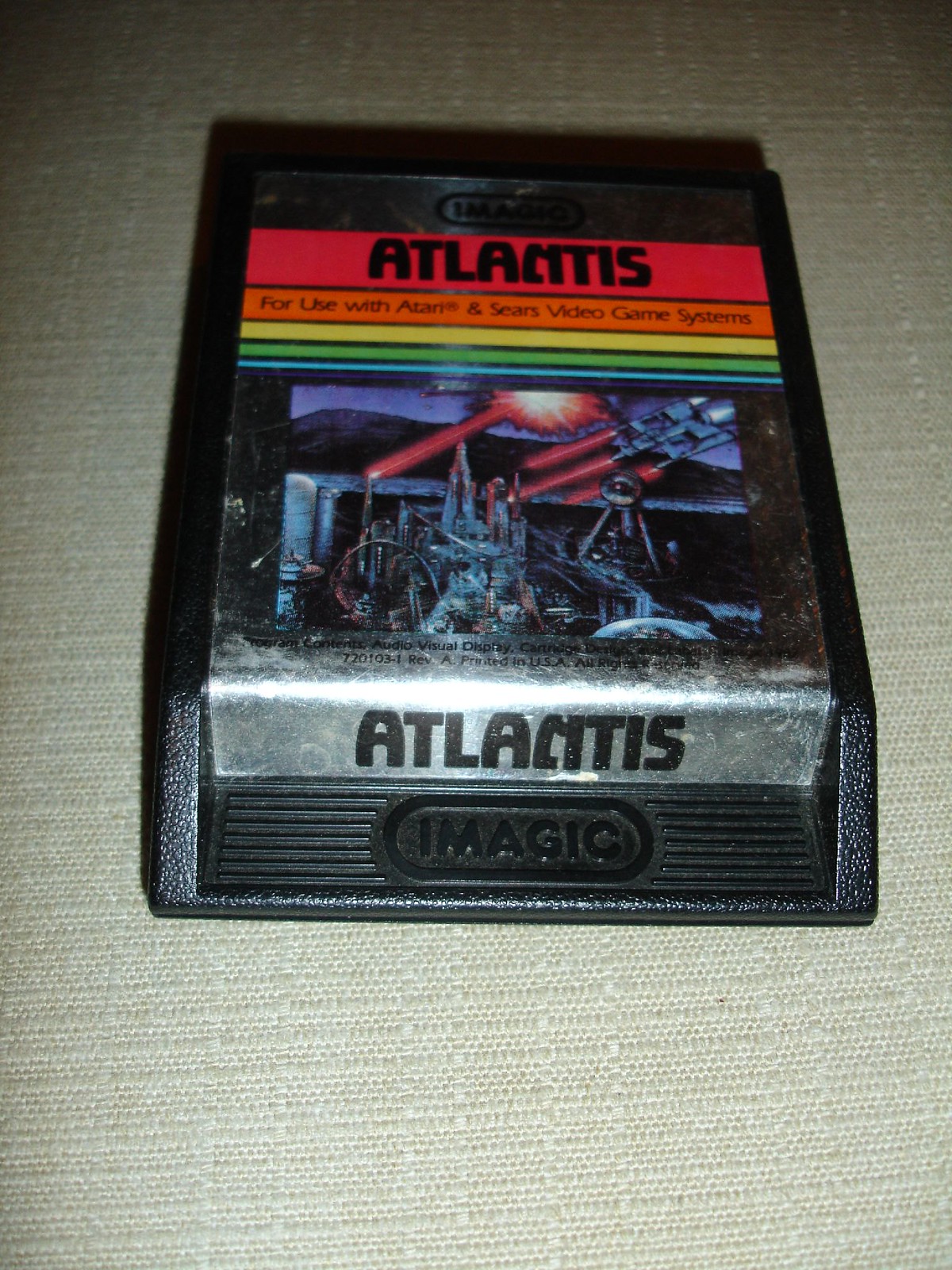Photograph of an "Atlantis" game cartridge designed for use with Atari and Sears video game systems. The cartridge features the word "Atlantis" boldly printed in red at the center. Around the label, vivid stripes in yellow, green, blue, and purple create a rainbow-like border at the top. The bottom section of the label showcases the "Atlantis" logo alongside the "IMAGIC" branding. The design includes a visually striking illustration of space drones, which adds to the sci-fi theme of the game. The cartridge itself resembles a classic cassette, with shadows near the top and more illumination towards the bottom, contrasting against a white cloth background.